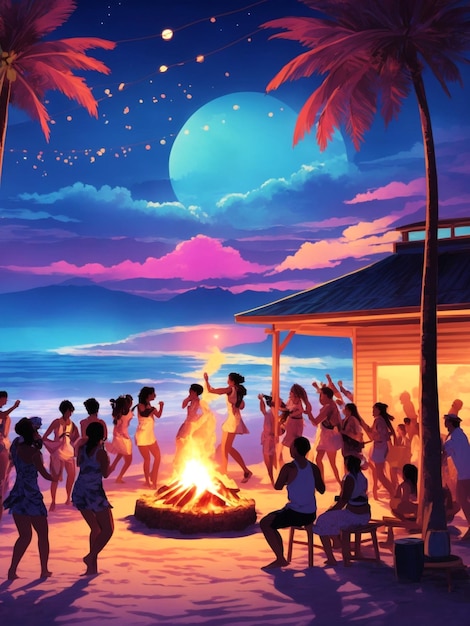The animated image depicts a lively island scene under a twilight sky. At the center, a bright orange bonfire blazes, surrounded by people dancing joyfully—some wearing dresses and others in tank tops. The ground is a beach with yellow sand leading up to the ocean's blue waves. Towering over the scene are palm trees with striking maroon leaves, adding a touch of exotic charm. In the backdrop, a large blue moon shines through pink and light orange clouds, casting a serene glow. To the right, there’s a small brown wooden building with a grey roof, beside which some wooden chairs are visible. Nestled in front of this building is another palm tree, completing the picturesque island gathering by the ocean.